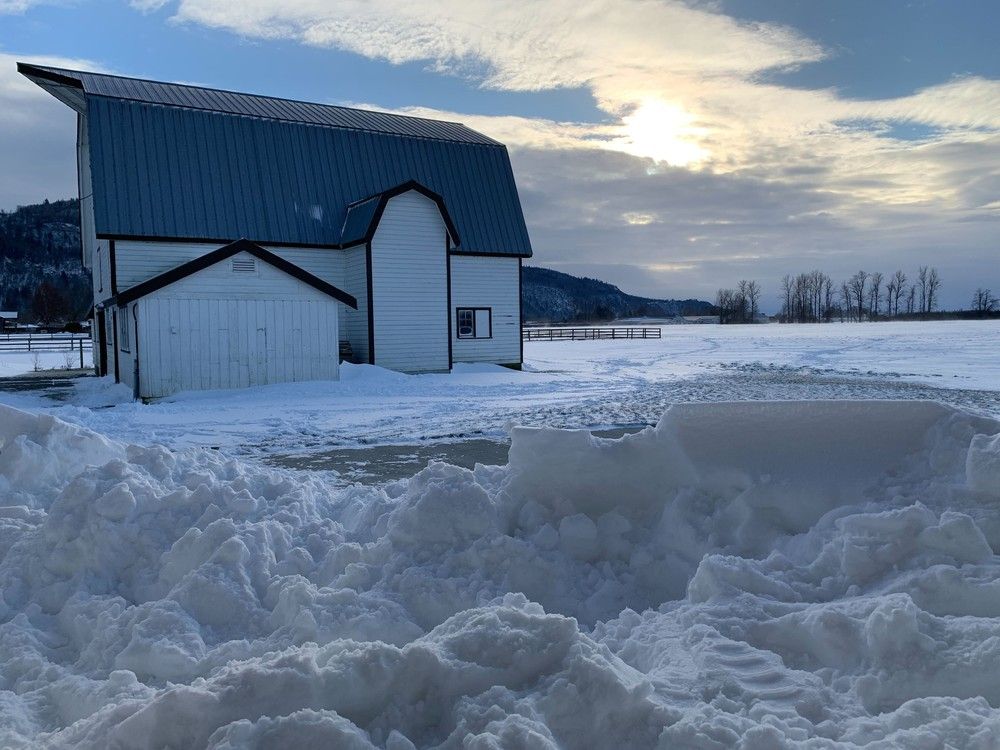This photograph captures a tranquil winter scene dominated by shades of white and gray. Set in a rural area, the landscape features a snow-covered field with patches of snow shoveled to the side in the foreground. A prominent white barn with a dark gray roof stands in the middle ground, its two-story structure displaying various shapes typical of barns, though it could also be mistaken for an old country church. The barn is complemented by a brown fence to its side, suggesting farmland usage. Bare trees frame the right side of the image, and the background reveals low-lying hills or a mountain, devoid of snow, under a sky partially obscured by dark gray clouds and a hazy sun. The faint hint of blue sky adds a subtle contrast, enhancing the serene and desolate beauty of this countryside winter morning.